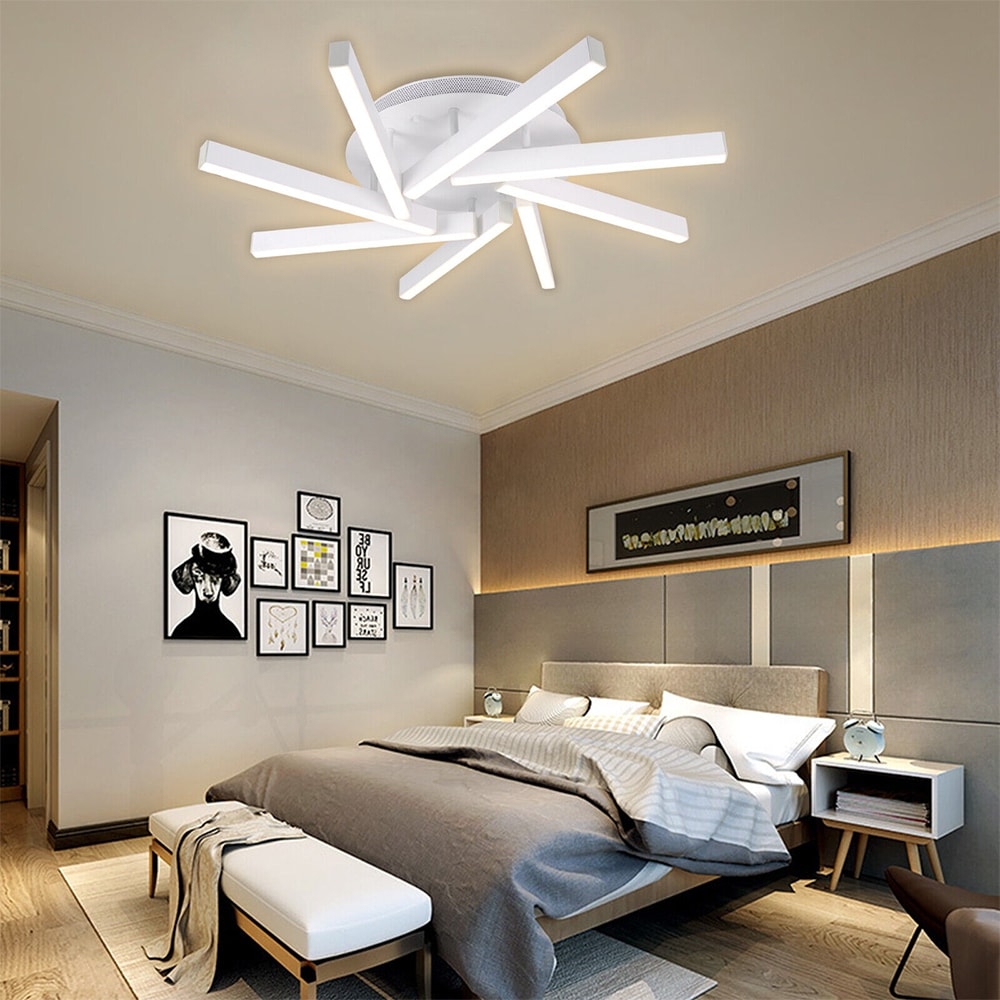The photograph captures an exceptionally modern and tastefully decorated bedroom with a neutral color palette. The room's walls combine light gray and beige tones, creating a soothing, elegant ambiance. The bed is positioned centrally against the wall and is draped with gray and white striped linens, complemented by three cushions against a matching gray headboard. On each side of the bed are minimalist white nightstands, each adorned with a traditional alarm clock.

Above the bed, an elongated rectangular piece of wall art in a gold frame draws attention, set against a darker gray section of the wall, contrasting with the tan wallpaper that occupies the upper half. Adjacent to the bed wall, a gallery wall showcases a collection of black-framed black-and-white drawings and prints, including text encouraging, "Be Yourself."

At the foot of the bed, a long white upholstered bench with golden legs serves as both a decorative and functional piece, with a throw or tan garment casually draped over it. The room’s light brown laminated wood floor adds warmth to the space.

Adding a unique touch, an abstract white ceiling fan stands out with its unconventional design, featuring thin white boards arranged in a round configuration, resembling a modern art installation. Overall, the room exudes a contemporary, serene vibe with its carefully curated details and harmonious color scheme.